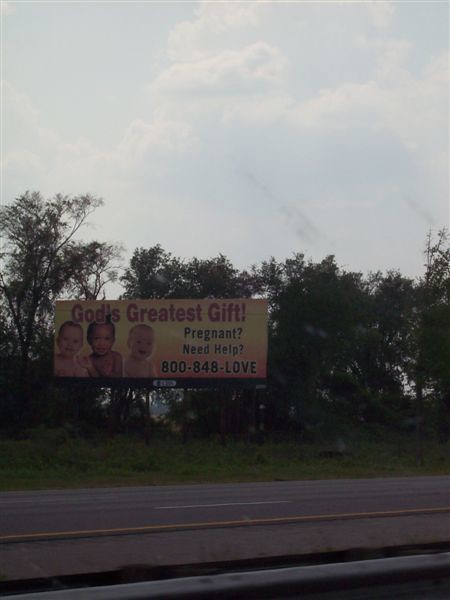The photograph captures a vibrant outdoor scene on a beautiful, clear blue day with scattered white clouds dotting the sky. In the distance, a lush line of trees stands tall, providing a serene natural backdrop. In the foreground, a prominent billboard commands attention. The billboard, set against a striking yellow and orange gradient background, bears a heartfelt message: "God's Greatest Gift, Pregnant, Need Help, 800-848-LOVE." Accompanying the text, in the left-hand corner beneath "God's Greatest Gift," are images of three children – two white infants and one African American baby, symbolizing innocence and diversity. Below the trees, a grassy area stretches out before a well-maintained road marked with a distinctive yellow centerline, indicating it's likely a highway. This impactful billboard serves as a poignant and supportive message from a pro-life organization, offering assistance and hope to those in need.